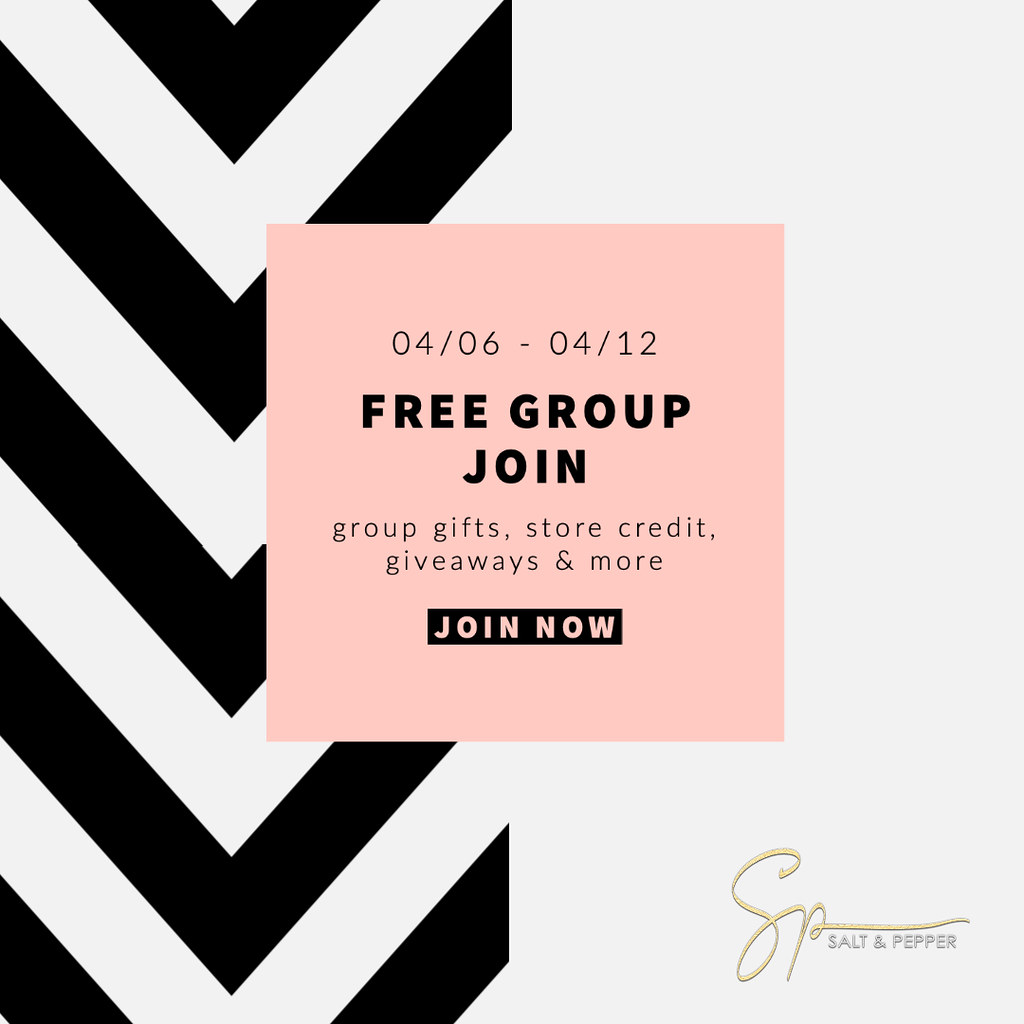The image is a promotional flyer with a split background. The left side features a repeating pattern of black, military-style arrows pointing downward, creating a striped effect, while the right side is a solid white block. In the center, there is a light pink square containing black text that reads "04-06 to 04-12" at the top. Below this, in black block capitals, it says "Free Group Join," followed by phrases in normal black text: "Group Gifts," "Store Credit," "Giveaways and More." There is also a separate block of black with pink text that states "Join Now." Positioned in the bottom right corner of the flyer, the branding appears with "SP" in a cursive font and a line through it, followed by "SALT AND PEPPER" in capital gray letters.